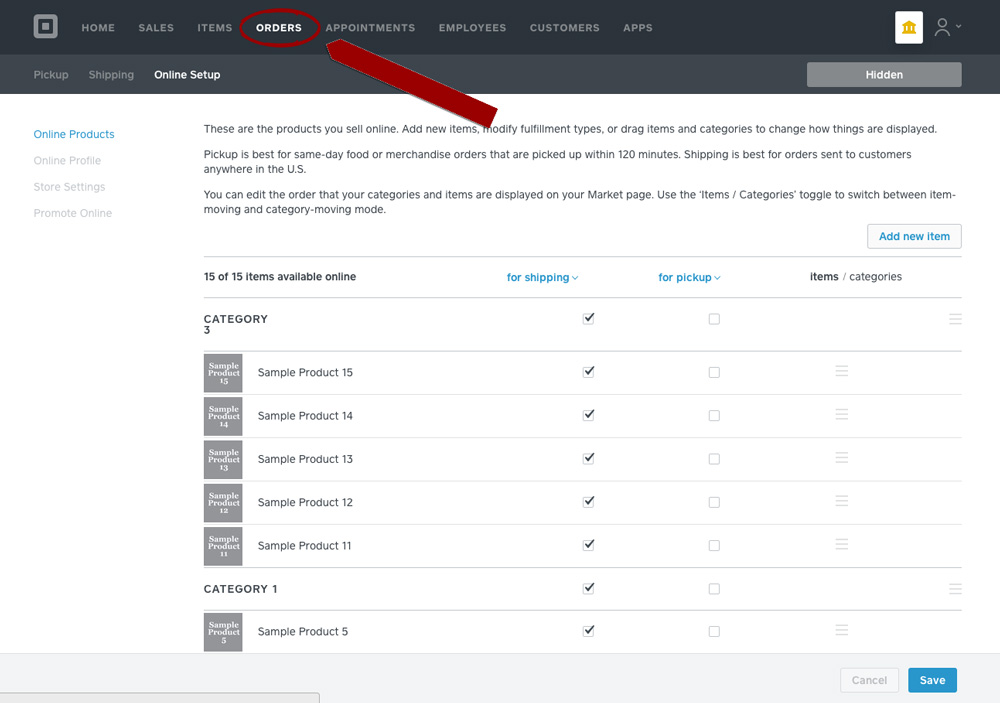The image showcases a website interface. The top section features a logo enclosed within a square, which itself is positioned inside a larger square. Below the logo, navigation links are clearly arranged, reading: Home, Sales, Items, Orders, Appointments, Employees, Customers, and Apps.

The main area of the page is labeled "Online Products," indicating that these are the items available for online sale. Instructions are provided on how to manage these products, including options to add new items, modify fulfillment types, or rearrange items and categories by dragging them. A note states that pickup is the preferred method for handling same-day food and merchandise orders.

The section displays various placeholder content, such as items labeled "Sample Product," numbered from 15 down to 5. These items are organized into different categories like "Category 1" and "Category 3." Each product has shipping options indicated by a checkbox labeled "Shipping," which are all marked as selected. There is also a "Pickup" checkbox next to each item, but none of these are checked.

Additionally, a visual cue in the form of a ribbon or arrow points toward the "Orders" link in the top navigation bar, highlighting its importance.